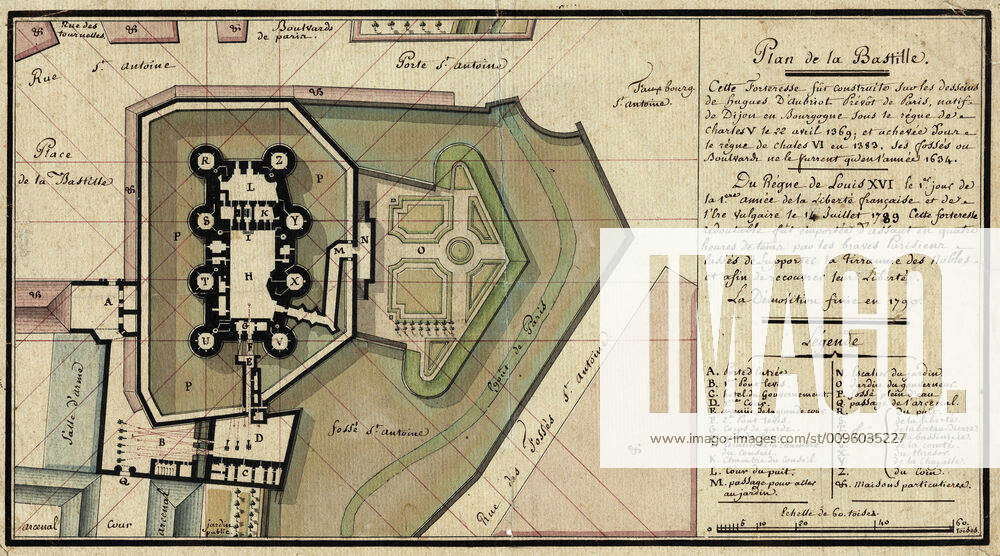The image showcases a detailed aerial blueprint in French, depicting a building complex, likely historical, resembling a fort or castle with multiple rounded turrets, surrounded by a garden area. Prominently featured is "Rue Saint Antoine" alongside the intricate layout. The blueprint is marked with a white watermark reading "Imago" and the website "www.imago-images.com/0096035227." Scattered across the map are various red-marked areas containing letters and numbers, likely corresponding to detailed descriptions on the right side. The right side features extensive cursive text, headlined by "Plan de la Bastille," providing further context and information about the structure and its surroundings.